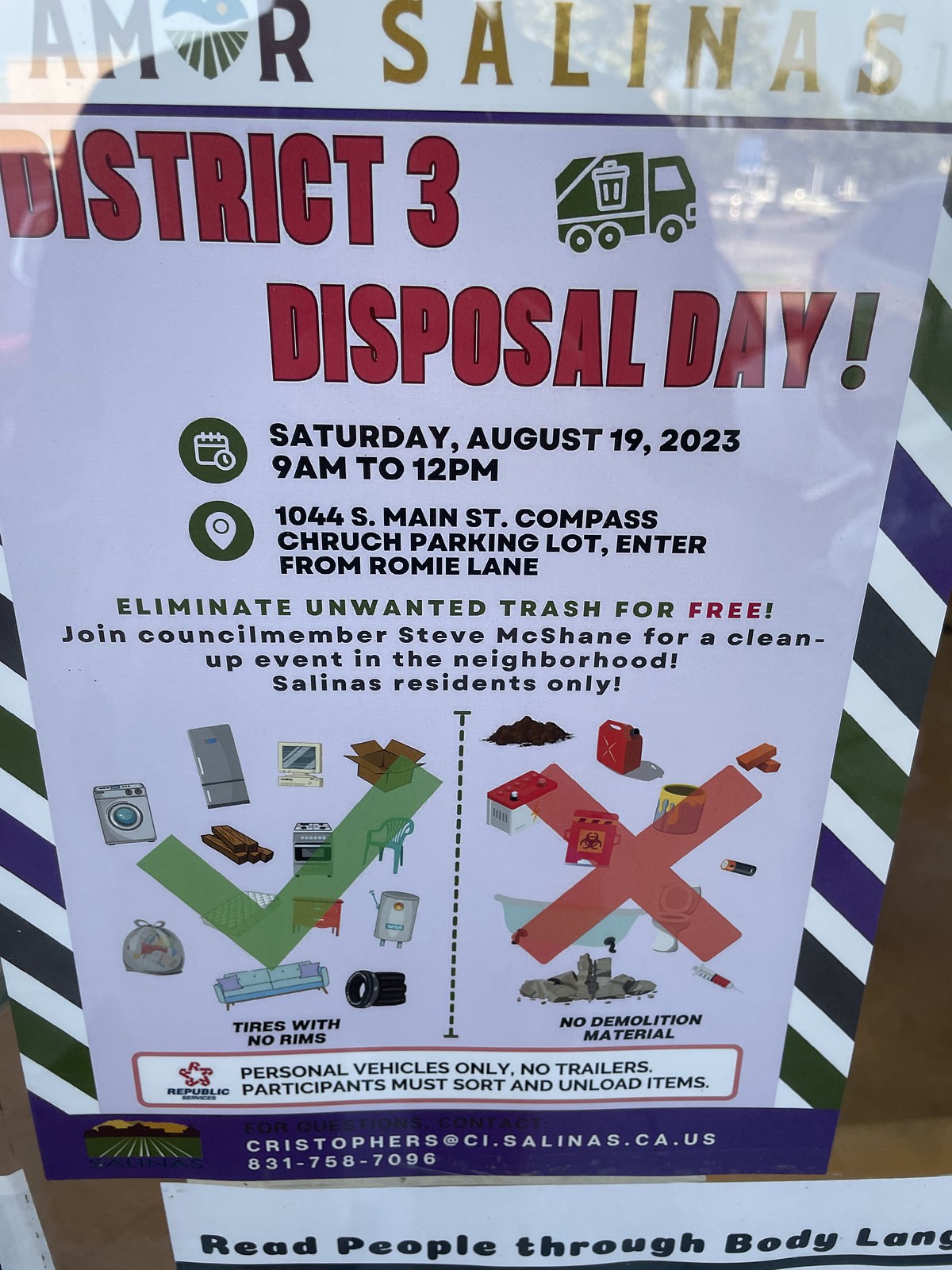The image is a full-color poster for the event "Armor Salinas District 3 Disposal Day," prominently featuring red, black, and yellow text. The main title, "District 3 Disposal Day," appears in bold red letters, while at the top, "Amor Salinas" is in all capital letters. The white background of the poster is encircled by diagonal blue and green stripes.

Below the title, the event's details are clearly displayed: it will take place on Saturday, August 19th, 2023, from 9 a.m. to 12 p.m., at 1044 South Main Street, Compass Church parking lot, with entry from Romy Lane. Important information emphasizes that this is a free cleanup event, exclusively for Salinas residents, hosted by Councilmember Steve McShane.

The poster contains visual aids: images of items that can be disposed of and those that cannot. On the left side, items with a green checkmark include plastic chairs, mattresses, couches, tires without rims, refrigerators, computers, and washing machines. On the right side, items with a red X indicating prohibited items include paint cans, batteries, bathtubs, syringes, toilets, and bricks. The notice also specifies that only personal vehicles are allowed, participants must sort and unload items themselves, and no trailers are permitted.

At the bottom, contact information is provided for further queries: Christopher at CI.Salinas.CA.US, phone number 831-758-7096. The poster design incorporates animation-style images and icons, making it both informative and visually engaging.